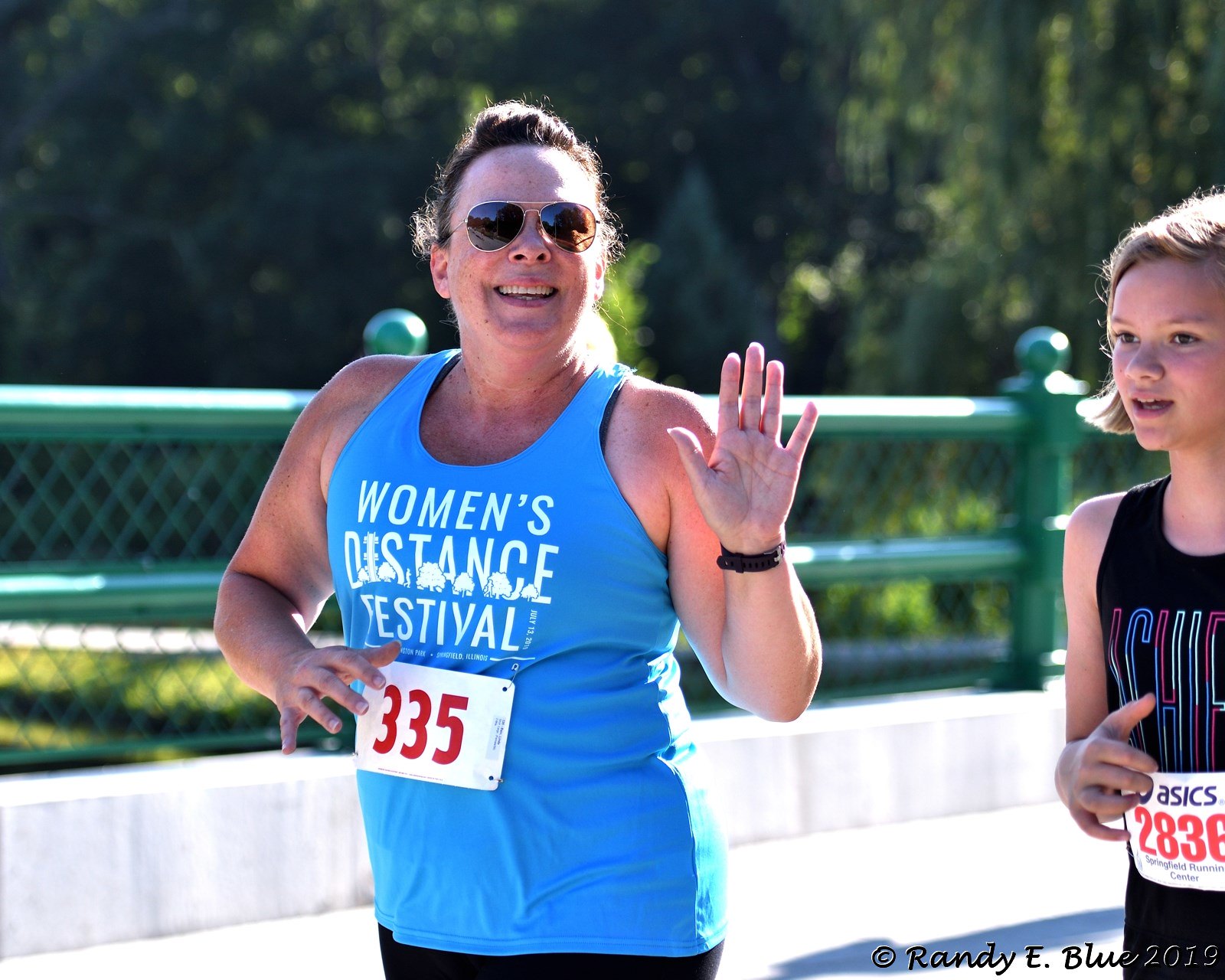In this vibrant photograph captured in 2019 by Randy E. Blue, a woman and a young girl are enthusiastically participating in a running race. The woman, likely in her 30s or 40s, is the primary focus. She has light skin and brown hair pulled back, and she is smiling broadly beneath her dark sunglasses. Dressed in a blue tank top that reads "Women's Distance Festival" in white lettering, she also wears black shorts or pants and a black-banded watch. Her race bib, numbered 335 in red, is prominently pinned to her front. Mid-stride, she waves at the camera with her left hand, while her right hand crosses her body. 

To her left, the right side of the image, a young girl with short blonde hair also runs enthusiastically. She sports a black tank top adorned with colorful, but indistinct lettering, and her race bib, numbered 2836 with "A6" in blue at the top, is secured to her chest. Her gaze is fixed straight ahead, possibly on the finish line.

The scene is set outdoors, likely along a street lined with a green fence, beyond which lush green grass and trees are visible, adding a refreshing backdrop to this lively moment of athletic camaraderie.